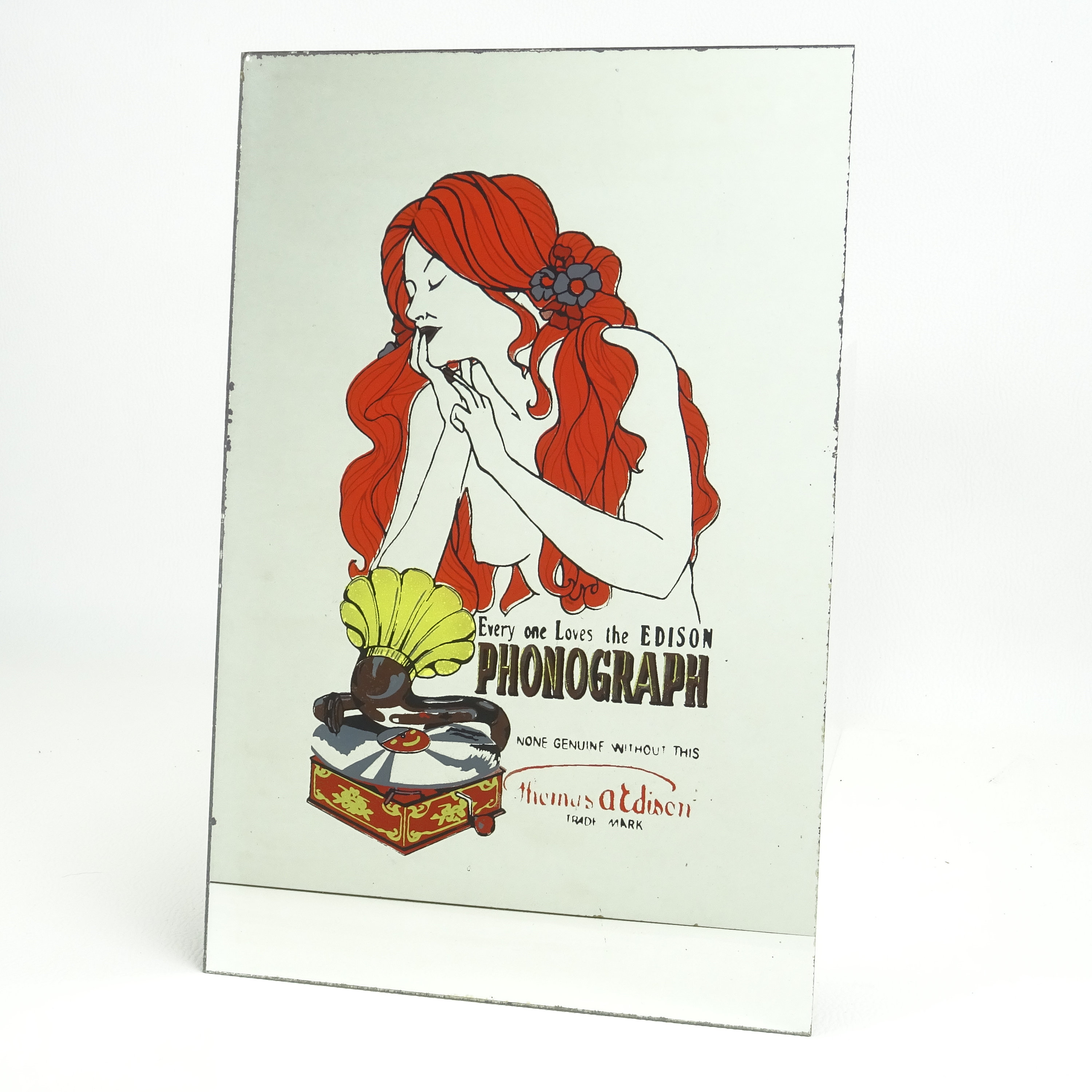The detailed image depicts a vintage Art Deco advertisement, most likely a reproduction, showcasing a painted illustration of a topless woman with very long, flowy red hair adorned with flowers. Her hair, tied back with additional flowers, cascades both in front and behind her, partially covering her body. She holds her chin with both hands, her eyes closed, and her face exhibits a look of wonder. The woman’s right breast is exposed. Below her, there is an antique red and gold phonograph with a long horn, characteristic of the late 1800s to early 1900s. To the right of the phonograph, bold text states, "Everyone Loves the Edison Phonograph," with the smaller subtext, "None genuine without this Thomas Edison trademark." The ad is on a white background, indicating it might be a modern product listing for purchase. The overall setting is bright and clear, although some of the red letters are slightly washed out and distorted.